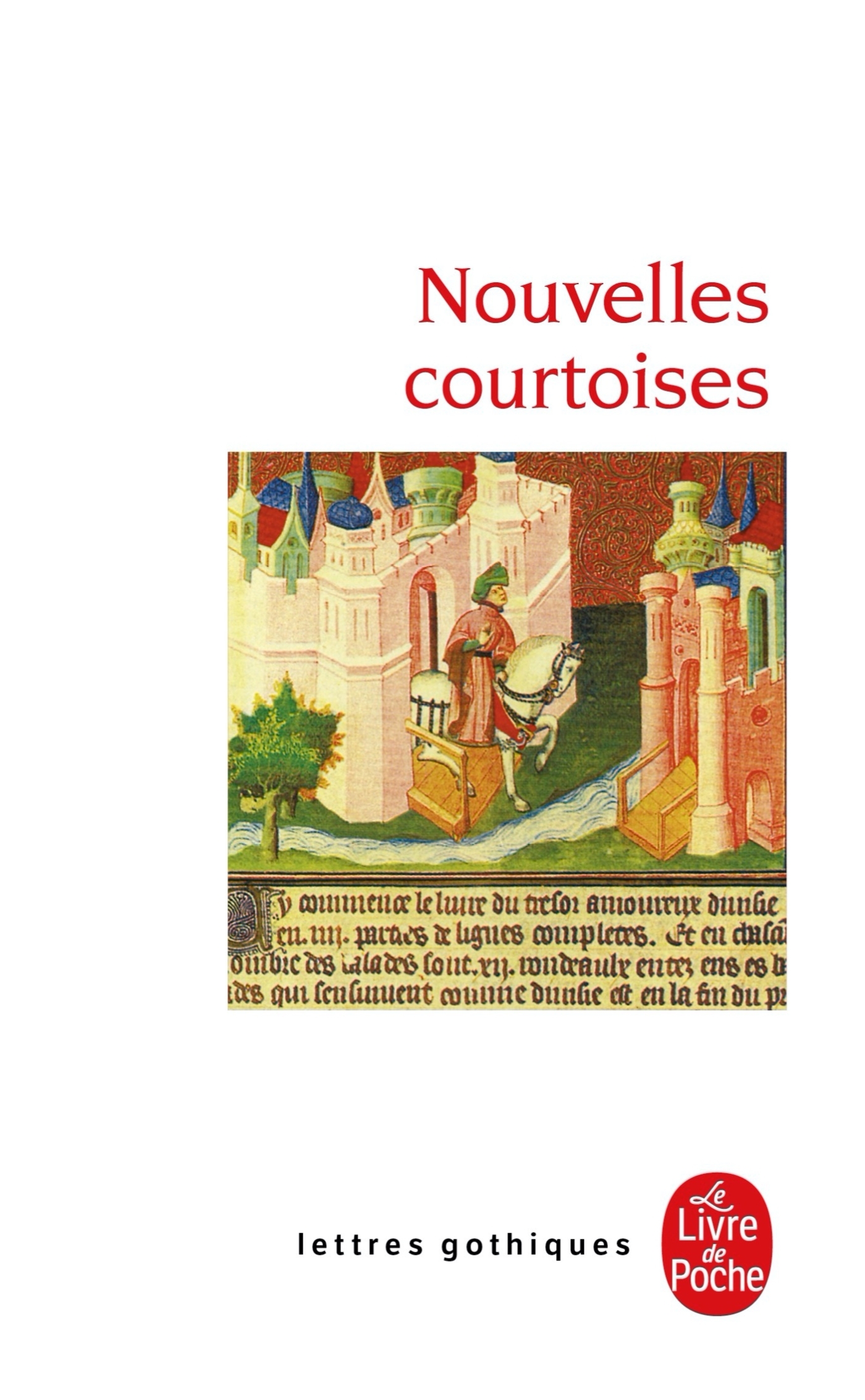The image is a detailed medieval illustration, possibly the cover of a book or a manuscript. It depicts a scene where a large figure, possibly a religious one, dressed in a pink robe and green turban, rides a white horse emerging from a white castle onto a wooden bridge. In the foreground, a green tree sits by a stream on the left. Across the stream, on the right, stands a red (or pink) castle adorned with green towers topped with blue roofs and featuring a wooden entrance. The scene is not to scale, as the rider is nearly the same height as the castles. 

At the top of the image, there are two lines of text in red, the first one reading "Nouvelles," and the second "Courtoises." Beneath the illustration, a manuscript section features black Latin-like text on a yellow background. Further down, more text in black letters reads "Lettres Gothiques," next to a red vertical oval with white letters inside possibly saying "Livre Poche."